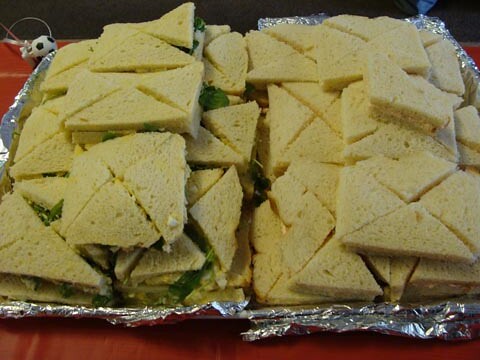This photograph captures a close-up view of a large aluminum foil-lined tray filled with numerous crustless sandwiches, stacked two to three layers high. The tray, somewhat wrinkled and crinkled at the edges, is placed on a reddish-brown, likely wooden or tiled, table surface. In the upper left corner of the scene, there's a small black-and-white soccer ball keychain. 

The sandwiches are meticulously cut into quarters, forming neat triangular shapes. On the left-hand side of the tray, the sandwiches appear to be filled with a leafy green vegetable, possibly lettuce or spinach, and possibly egg or chicken salad, based on the visible yellow and green fillings. On the right-hand side, the sandwiches feature what seems to be cheese and perhaps bologna, given their light-yellow interior. The sandwiches are organized by type, forming distinct piles. 

No serving utensils or toothpicks are present, suggesting these finger foods are ready to be grabbed directly from the tray, likely at a casual gathering such as a potluck or picnic.